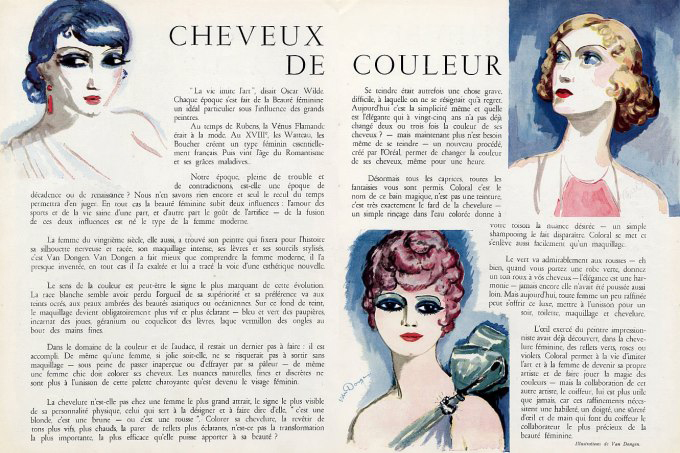The old magazine features an article titled "Cheveux de Couleur," translating to "Colored Hair" in French, with the title prominently displayed in bold black letters against a very light pink background. Spanning two pages, the lengthy article is divided into three columns, with one column almost filling the left page and two columns occupying the right. The article is accompanied by three distinct illustrations of women in older fashion hairstyles and attire.

The top left illustration depicts a woman with striking blue hair, heavily caked-on grey eyeshadow, thick false eyelashes, long skinny eyebrows, red pendant earrings, and pink lips. She appears to be wearing a white sleeveless top. The top right illustration shows a woman with short, curly blonde hair, blue eyes, and horrible eye makeup, including red lips, and she is dressed in a pink top. The bottom middle illustration is particularly striking, featuring a woman with disproportionately large eyes, long skinny eyebrows, heavily applied turquoise eyeshadow, red lips, and short reddish hair styled in curls piled up on her head. She is adorned in a turquoise outfit. Each woman gazes out with a peculiar charm, echoing the fashion and makeup styles that seemingly harken back to the 1920s.